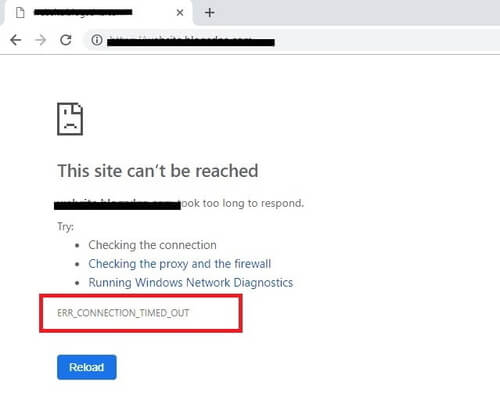A person is using the Google Chrome browser and has entered a URL, which is visibly censored with a black bar, preventing the URL and the tab information from being seen. The webpage displays a generic error message, featuring a "sad piece of paper" icon and stating, "This site can't be reached." The error message explains that the address took too long to respond and suggests troubleshooting steps such as checking the connection, proxy, and firewall settings, or running Windows Diagnostics. At the bottom, it specifies "ERR_CONNECTION_TIMED_OUT" and includes a blue "Reload" button. Additionally, a red outline highlights the "ERR_CONNECTION_TIMED_OUT" portion of the message. The reasons for the URL censorship and the connection issues are unclear, leaving room for ambiguity about whether the problem lies with the website or the user's setup.